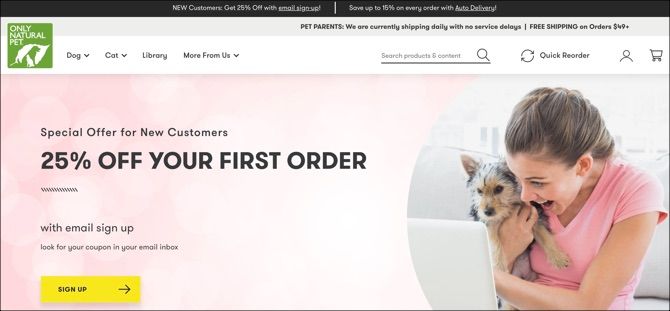The image depicts a vibrant pet care website centered around eco-friendly products. Prominently positioned on the left is the site’s heading, "Only Natural Pet," accompanied by a green logo that merges the shapes of a leaf with the outlines of a dog and a cat, symbolizing the company's commitment to environmentally conscious pet care solutions.

At the top navigation toolbar, users can find specific categories like "Dog" and "Cat," along with additional sections such as "More From Us" and "Pet Parents." There’s also a prominent announcement: "We are currently shipping daily with no service charge. Free shipping on orders."

Below the toolbar, the main area of the website features a cheerful young woman wearing a pink top, joyfully holding her dog while both look at the computer screen, suggesting they are exploring products together. To the left of the woman, a highlighted pink banner promotes a special offer: "25% off your first order for new customers with email sign-up. Receive your coupon in your email inbox."

This detailed and user-friendly website appears to specialize in providing natural pet food, toys, and other pet care products.